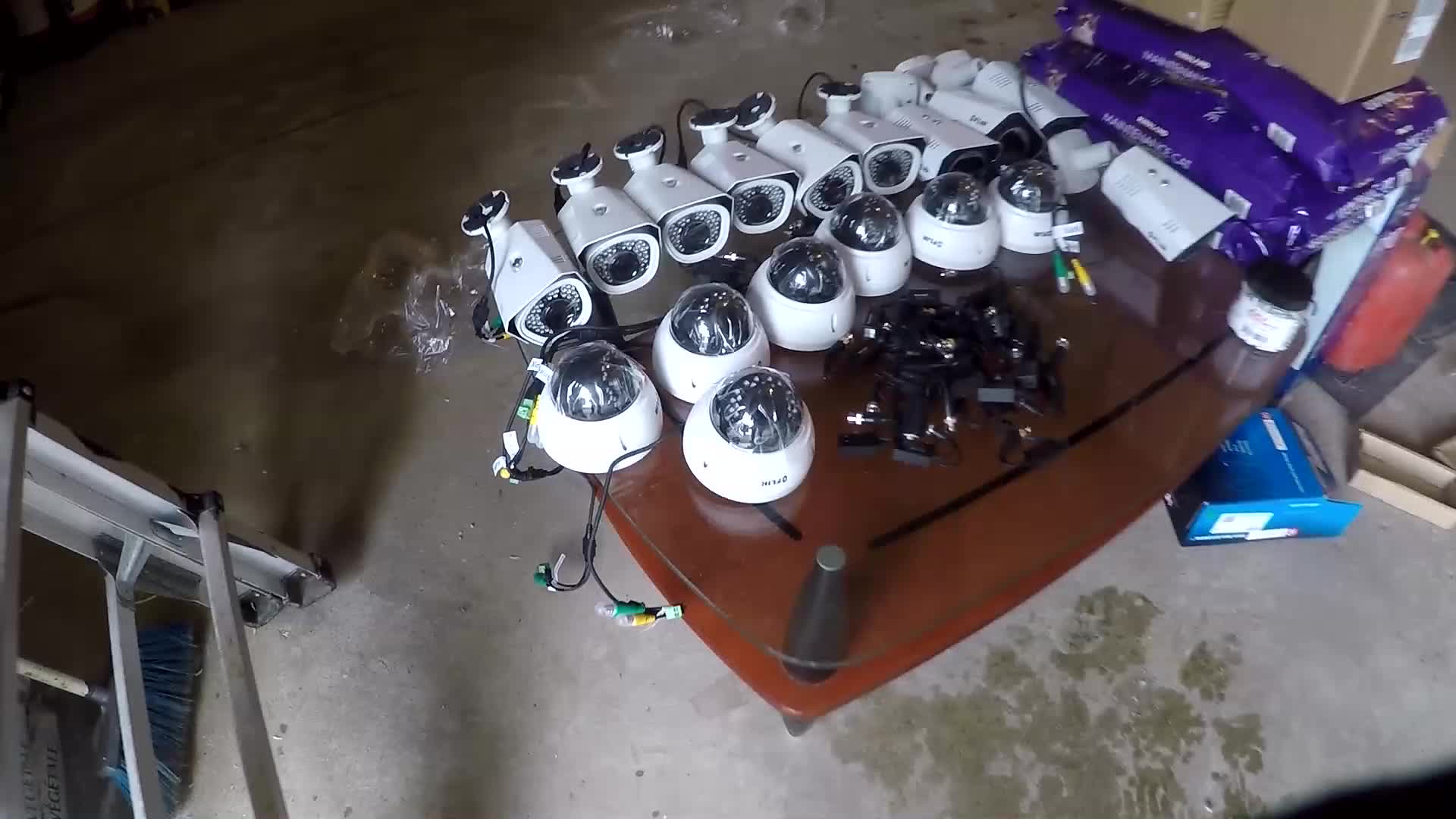The photograph depicts a cluttered scene in what appears to be a basement or garage. A glass-top table with a brown wooden base sits on a concrete floor, surrounded by random spots and minimal clutter. The table holds two distinct types of security cameras. In the center are several dome cameras, featuring white round bases and black glass bubbles, typically installed on ceilings to appear inconspicuous. Scattered around these dome cameras are black mounting brackets and a few silver screws. Toward the edge of the table, a row of rectangular, more conspicuous security cameras can be seen, characterized by their white housing and black lenses with cables protruding from them. The image, of digital camera quality, appears slightly out of focus. Additional items include two stacked blue plastic bags labeled "maintenance care" to the right, and a red gas can and a ladder visible in the bottom left corner of the photograph.